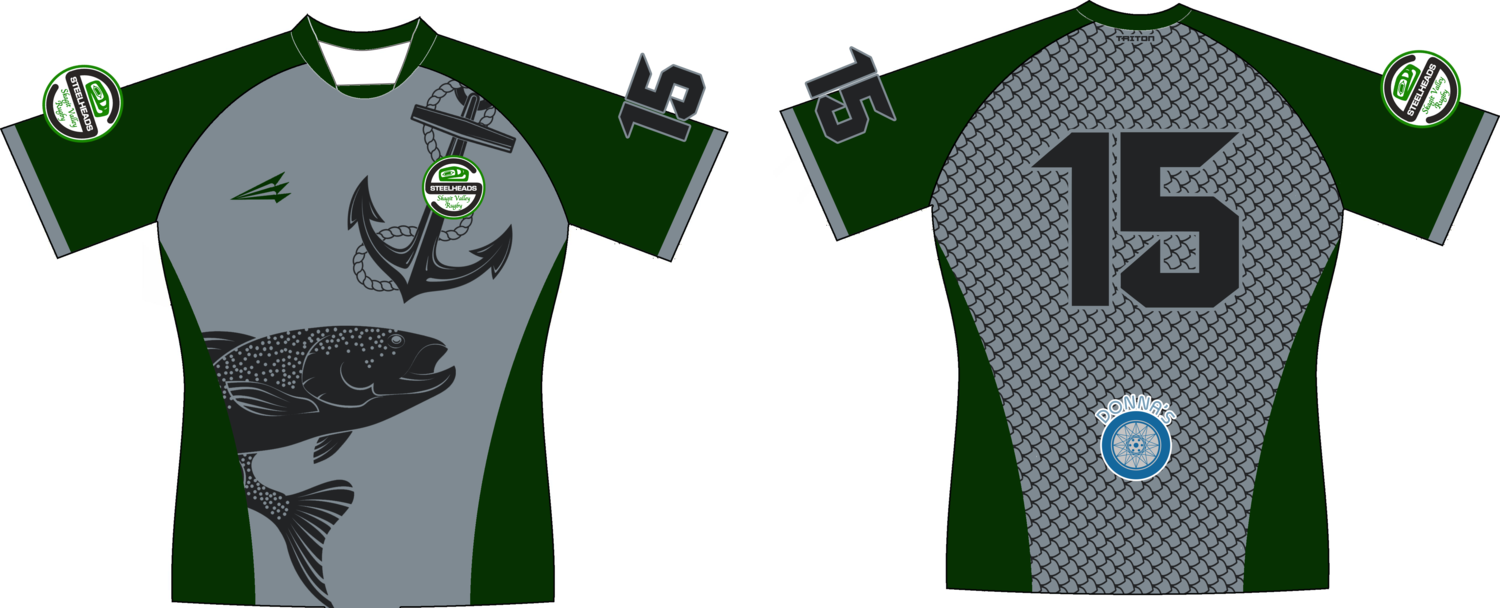This image features a computer-generated digital mock-up of a sports jersey shown in landscape orientation, with the front view on the left and the back view on the right, both set against a white background. The jersey predominantly features a dark green and medium gray color scheme. 

The front of the jersey, on the left side of the image, displays a medium gray body with dark green stripes on the sides and green short sleeves. It has a squarish neckline. Over the right chest area, there's a large dark gray boat anchor with a rope, and across the stomach area is a big, dark gray fish resembling a trout or steelhead. The left sleeve bears a circular white patch with a tiny, unreadable image, and the right sleeve prominently displays the number 15 in black.

The back of the jersey, on the right side of the image, mirrors the dark green sleeves and neckline but shifts to a gray center with black diagonal lines forming a scale-like pattern. The black number 15 appears prominently in the center. Below this number, there is a light blue circle with white inside, displaying tiny, unreadable writing possibly suggesting "Donna's." On the left sleeve is a black number 15, while the right sleeve shows the circular white patch with the steelhead-like badge emblem.